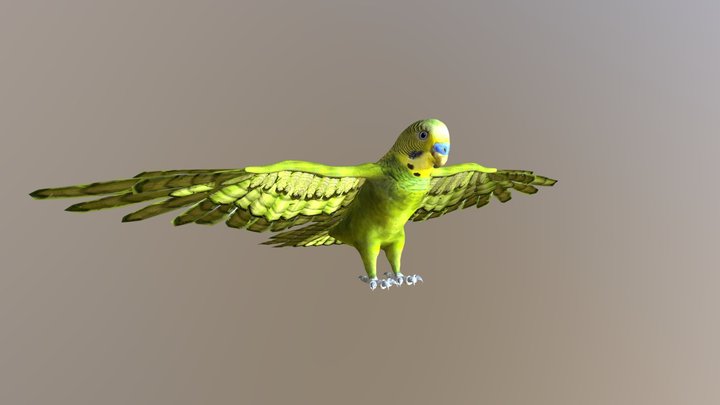This is a detailed illustration of a tropical parrot in mid-flight against a light gray background. The parrot, primarily lime green with a mix of yellow around the neck, has its wings fully extended, showing black spots along the edges. The beak is light brown, featuring blue coloration near the tip, and the eyes are circular and black. The parrot's legs and white talons are visible, with a slight greenish-yellow hue on the body and legs. The bird appears to be flying towards the bottom right, presenting a dynamic side view. The detailed textures and colors suggest that this may be a CGI or drawing rather than a real photograph.